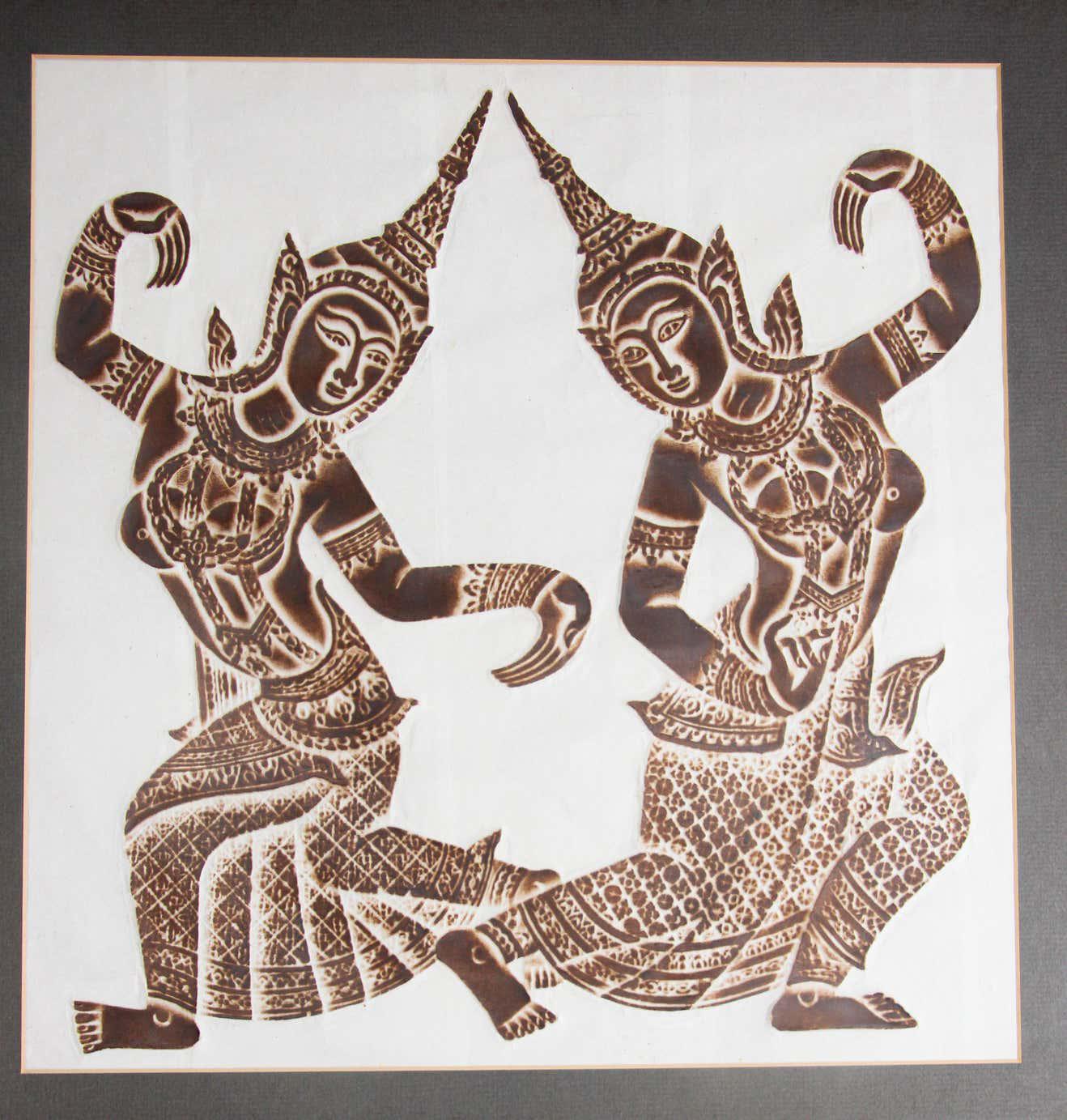The image is an old art piece encased in a frame, which could either be grey or set against a grey wall. The inner frame has a peachy hue, surrounding the artwork that stands out against a white or off-white background. The painting, rendered on what appears to be white paper, is meticulously designed using dark brown hues and negative space to emphasize the white background.

It depicts two women in a dance pose, artistically crafted and revealing a surprising level of detail for something so ancient. Both women are adorned in nearly identical, very see-through netting costumes with intricate patterns on their long skirts. They wear tall, pointed headdresses and elaborate necklaces or neck pieces that blend into their tops. Their hands are elegantly curved around each other, enhancing the sense of movement.

The women are positioned so that the one on the left looks towards the right, and the other on the right gazes leftward, creating a balanced and harmonious composition. The absence of an artist's signature on the painting only adds to its mysterious allure and historic elegance.